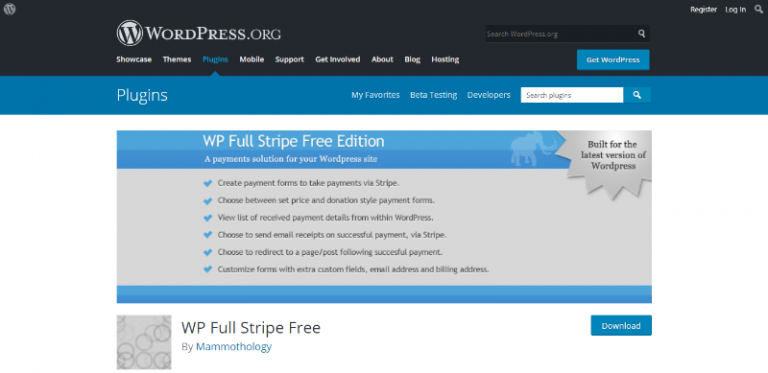This widescreen landscape screenshot showcases the WordPress.org website. At the top, a sleek black banner features the WordPress.org name in white font, accompanied by the WordPress logo—a black "W" encased within a white circle. Directly below this, a navigation menu offers quick access to sections labeled Showcase, Themes, Plugins, Mobile, Support, Get Involved, About, Blog, and Hosting. Positioned to the right is a prominent "Get WordPress" button, with a Search WordPress.org bar neatly situated above.

In the upper right-hand corner, options for Register, Login, and Search are readily accessible. Just below, a vibrant blue banner highlights the Plugins section, including tabs for My Favorites, Beta Testing, and Developers, along with a Search Plugins bar on the right.

Beneath this, a detailed box introduces the "WP Full Stripe Free Edition," a versatile payment solution for your WordPress site. The description elaborates on its features: creating payment forms to process payments via Stripe, offering both set price and donation-style payment options, viewing a comprehensive list of receipt payment details within WordPress, sending email receipts for successful payments through Stripe, redirecting users to a specific page following payment, and customizing forms with additional fields like email and billing addresses. A Download button is prominently displayed, inviting users to install this software.